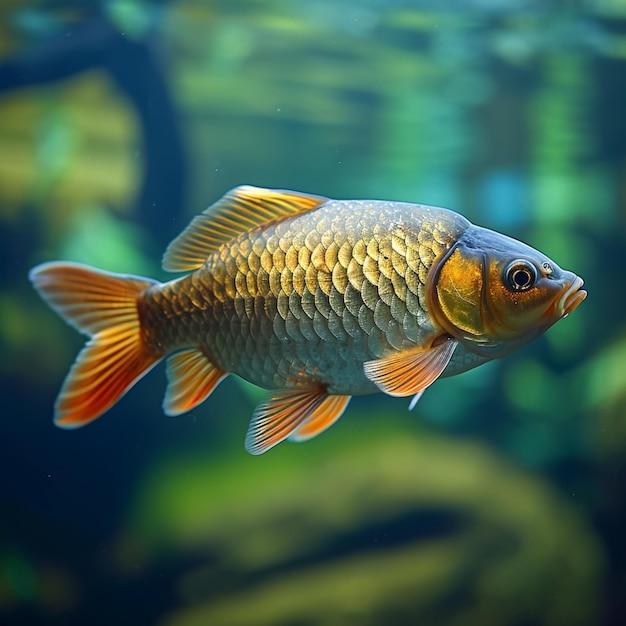This vivid close-up photograph highlights a goldfish swimming to the right, with the fish in sharp focus against a blurred, mottled background in shades of blue, green, and yellow, possibly reflecting aquarium glass. The goldfish showcases a striking array of colors: its body is adorned with shimmering golden scales, which transition to a silvery hue on the belly. The head is darker brown, with a black-tinged forehead, and a pronounced black eye. The goldfish has a total of six fins: two pectoral fins near the sides of its body, two ventral fins near the stomach, one anal fin close to the genital area, and a dorsal fin on top. The dorsal fin is a whitish-yellow, while all the bottom fins and the tail fin display a rich dark orange with golden stripes. Intricately lined fins enhance the elegance of this serene aquatic creature swimming through the softly lit water, with light reflecting off its upper body, lending a slight bluish tint to its top side.